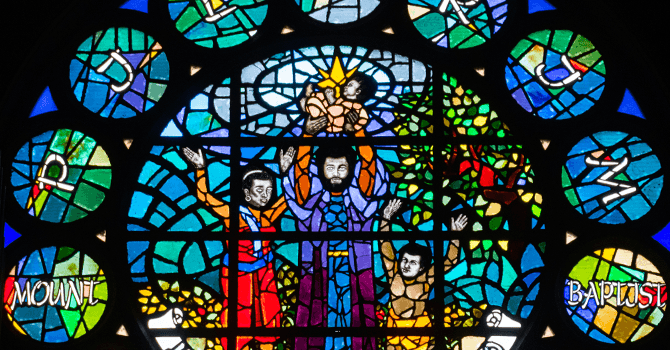The image depicts an intricate and vivid stained-glass window set in an arched shape. Central to this elaborate glasswork is a circular window surrounded by several multicolored rings, adorned with geometrical, irregular quadrilateral patterns. The central image portrays a father, wearing a blue and purple robe with orange sleeves and a red collar, joyously lifting his baby. To his left stands his wife, dressed in red and orange, and to his right is their child, clad in brown and raising their hands.

Prominently, the stained glass is inscribed with various letters and phrases. On the left side, the word "Mount" is written in white, while the right side features "Baptist." Other noticeable letters include P, J, another J, E, R, and M, suggesting a potential religious or communal message. The overall color palette of the glass integrates hues of blue and green, contributing to the scenic architectural setting that likely belongs to a church.